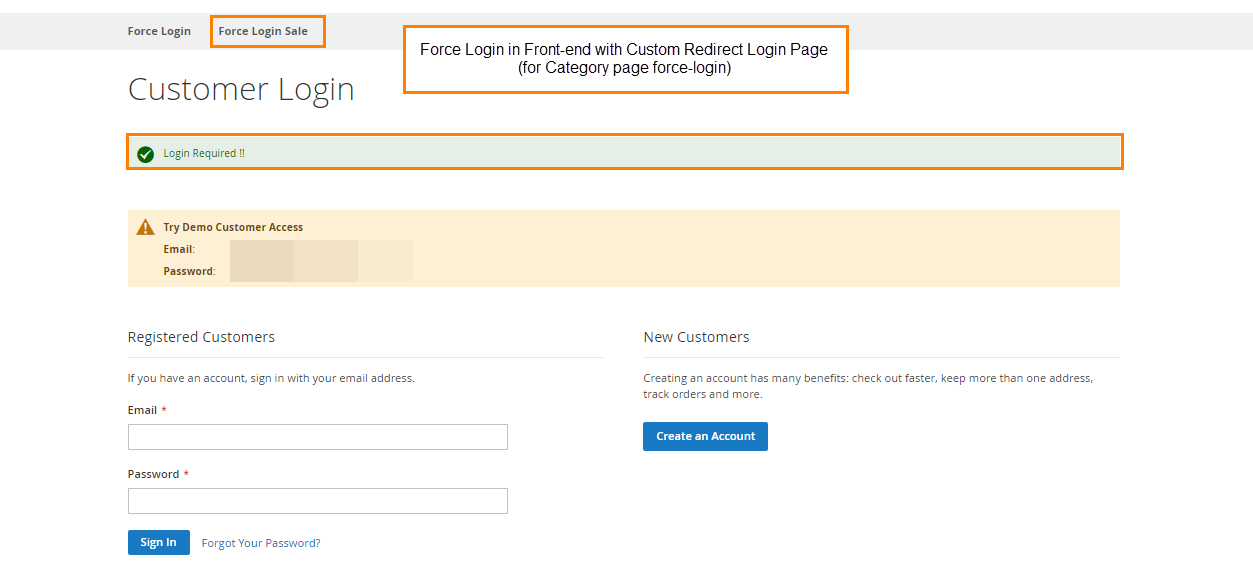Screenshot of a website's login page:

At the top left corner of the webpage, there is an option labeled "Force Login" encased in a red rectangle. Adjacent to this, on the right, is another red-encased label stating "Force Login Sale." In the center-top part of the page, a prominent notification reads: "Force login in front end with custom redirect login page for category page force login."

Further along the top left, there is a header that reads "Customer Login" with a green notification underneath in a red-highlighted box, stating "Login required." Below this, there is a yellow notification saying "Try demo customer access." This section appears to contain blurred-out trial email and password information.

Going down to the bottom left, there is a section titled "Registered Customers." It prompts users to sign in with their email address, providing text fields for email and password input, followed by a "Sign In" button.

To the right of the Registered Customers section, there is a "New Customers" area with a prominent "Create an Account" button, encouraging new users to sign up.